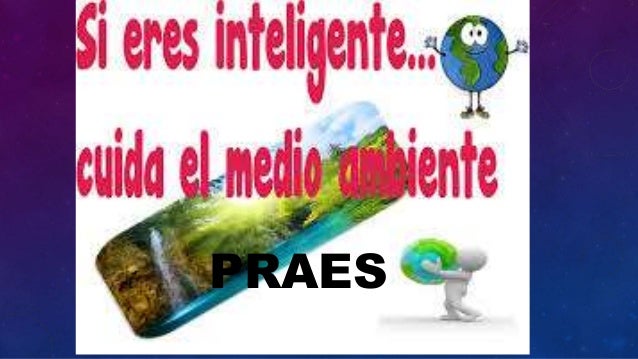The image features a vibrant, computer graphic scene set against a white background. Dominating the composition is a playful animated globe character with arms, legs, and googly eyes, accompanied by a neutral white figure holding the Earth. Above, red text boldly states, "Si eres inteligente... cuida el medio ambiente," which translates to "If you are intelligent... take care of the environment." Below, the acronym "PRAES" appears in bold, black, capital letters. A prominent diagonal photograph of a serene landscape—depicting a waterfall cascading into a turquoise-green lake, framed by trees, a blue sky with scattered white clouds, and bordered with a gradient from purple to blue—adds to the visual complexity. The left and right sides of the image are bordered asymmetrically with thick gradient blue coloring, thinner on the left and thicker on the right, adding a dynamic frame to the entire composition.